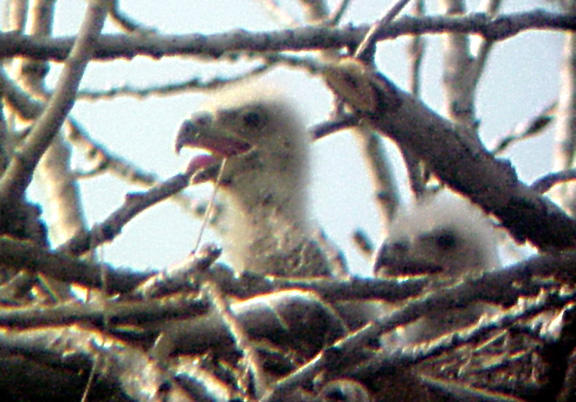The image captures a slightly blurry, close-up view of a nest occupied by two baby birds, possibly baby eagles or hawks, indicated by their sharp, slightly curved beaks. Both birds have dull white to gray feathers on their heads, and one bird is prominently sticking its head up with its mouth open, displaying its tongue, possibly awaiting food. The other bird is nestled lower in the nest with its mouth closed. The nest itself is constructed from various-sized branches and twigs, predominantly gray and arranged in a dense, heavy structure, suggesting the nest belongs to a large bird species. The background features a clear blue sky with no clouds, and faintly visible white trees, which could be birch, framing the scene.